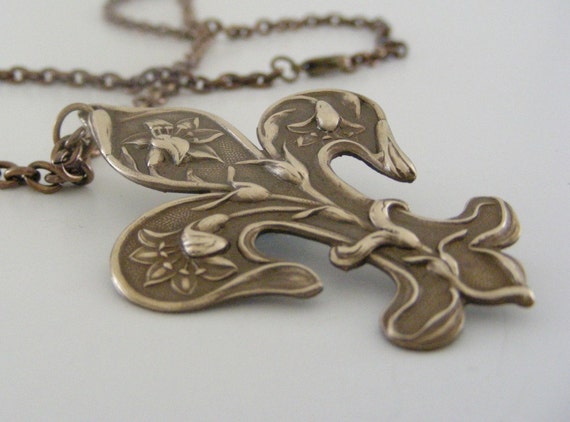This close-up photo captures an ornate fleur-de-lis necklace, prominently displayed against a pale purple background. The necklace features a finely detailed fleur-de-lis charm crafted from a bronzy silver metal with a patina finish. Each arm of the fleur-de-lis design is intricately adorned with flowers and intertwining vines, showcasing its delicate craftsmanship. The chain, which is slightly out of focus as it trails towards the upper left, is composed of small links in a matching bronzy brownish color, complementing the charm. This composition highlights the charm's intricate details and the cohesive coloration of the entire piece.